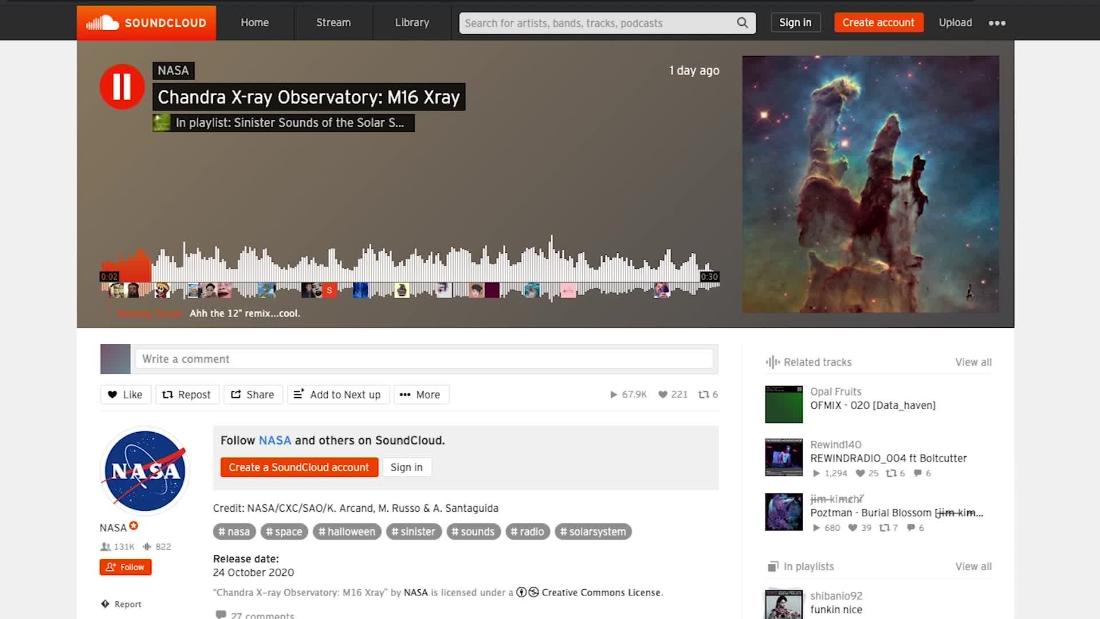A vibrant screenshot from SoundCloud captures a colorful printout featuring the SoundCloud logo and various navigation options—Home, Stream, Library, Search, Sign In, Create Account, and Upload—arrayed across the top right. The main focus centers on a playlist titled "Sinister Sounds of the Solar" by NASA Chandra X-ray Observatory, specifically highlighting the "M16 X-ray" track posted one day ago. The playlist's intriguing theme is matched by a visually striking background image resembling a colorful, monster-filled gaming scene. The presence of a rhythmic white icon indicates that music is currently playing. Below, users are invited to leave a comment in a designated "Write a comment" section. Additional details reveal prompts to follow NASA and other creators on SoundCloud. The official NASA logo, bearing the signature blue, red, and white colors, appears alongside credits for NASA employees and multiple clickable options. The release date of the featured content is marked as October 24, 2020. To the right, an assortment of related tracks is displayed with an option to view the entire list.